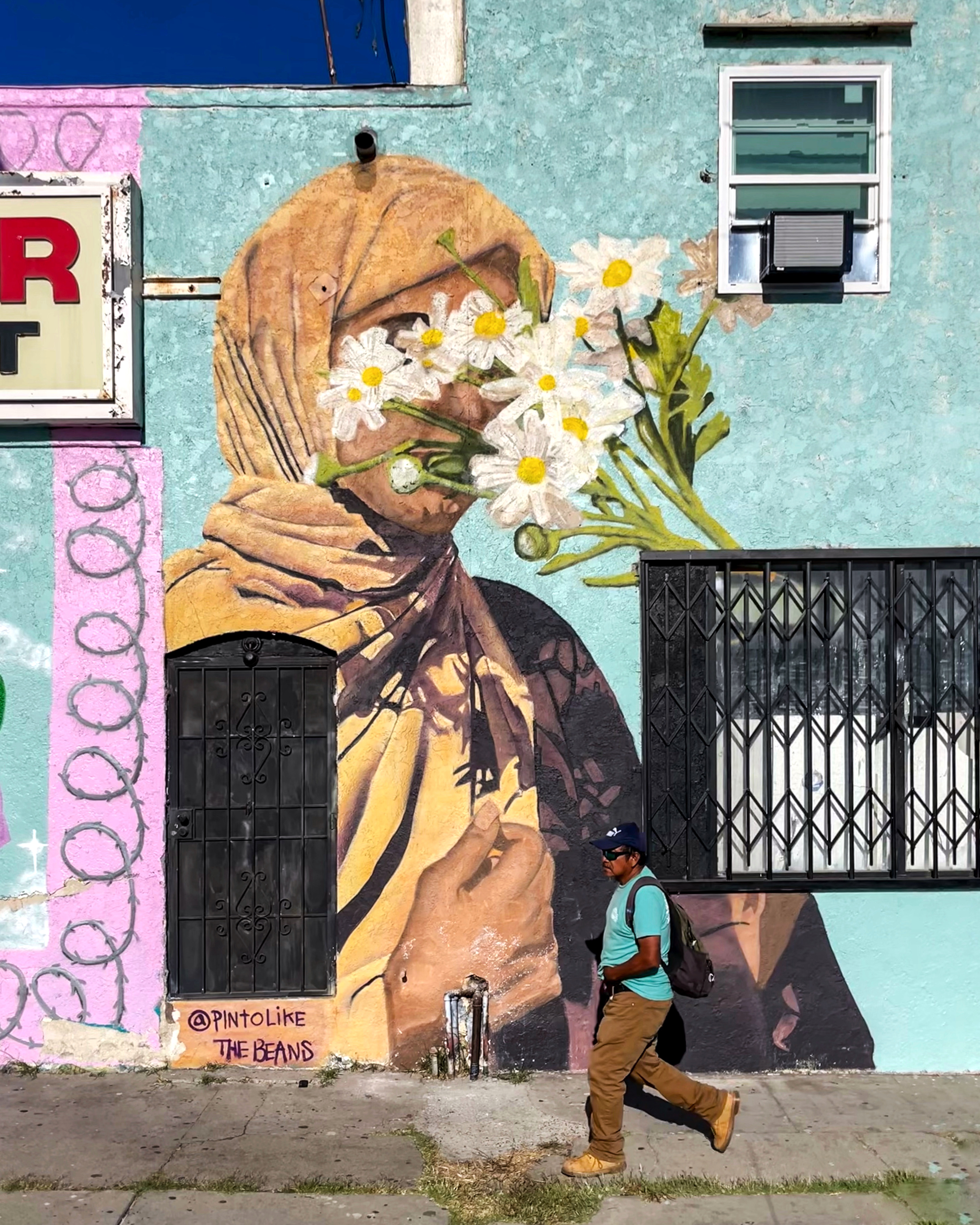The image is a color photograph taken outdoors, depicting a large mural painted on the side of a two-story building. The mural features a woman, likely of Middle Eastern descent, wearing a tan-colored hijab that envelops her head and shoulders. Her face is obscured by a bouquet of white daisies with yellow centers, giving the impression that she is holding or smelling them. The backdrop of the mural is primarily light blue, transitioning to dark blue at the top left, and includes various elements such as a pink rectangle with barbed wire.

The mural cleverly incorporates elements of the building's architecture. To the top right is a smaller window, partially open with a black air conditioning unit sticking out. Below the woman’s depicted torso, there is another window with decorative black iron security bars. The artist's name, "Pinto-like the beans," is written at the base of the mural.

In the foreground, a sidewalk stretches across the image, where a man of color is seen walking. He is wearing a medium blue shirt, brown pants, a black backpack, and a baseball cap. The pavement exhibits cracks with grass sprouting through, adding to the texture of the scene. The man appears to be in motion, adding a dynamic element to the photograph.